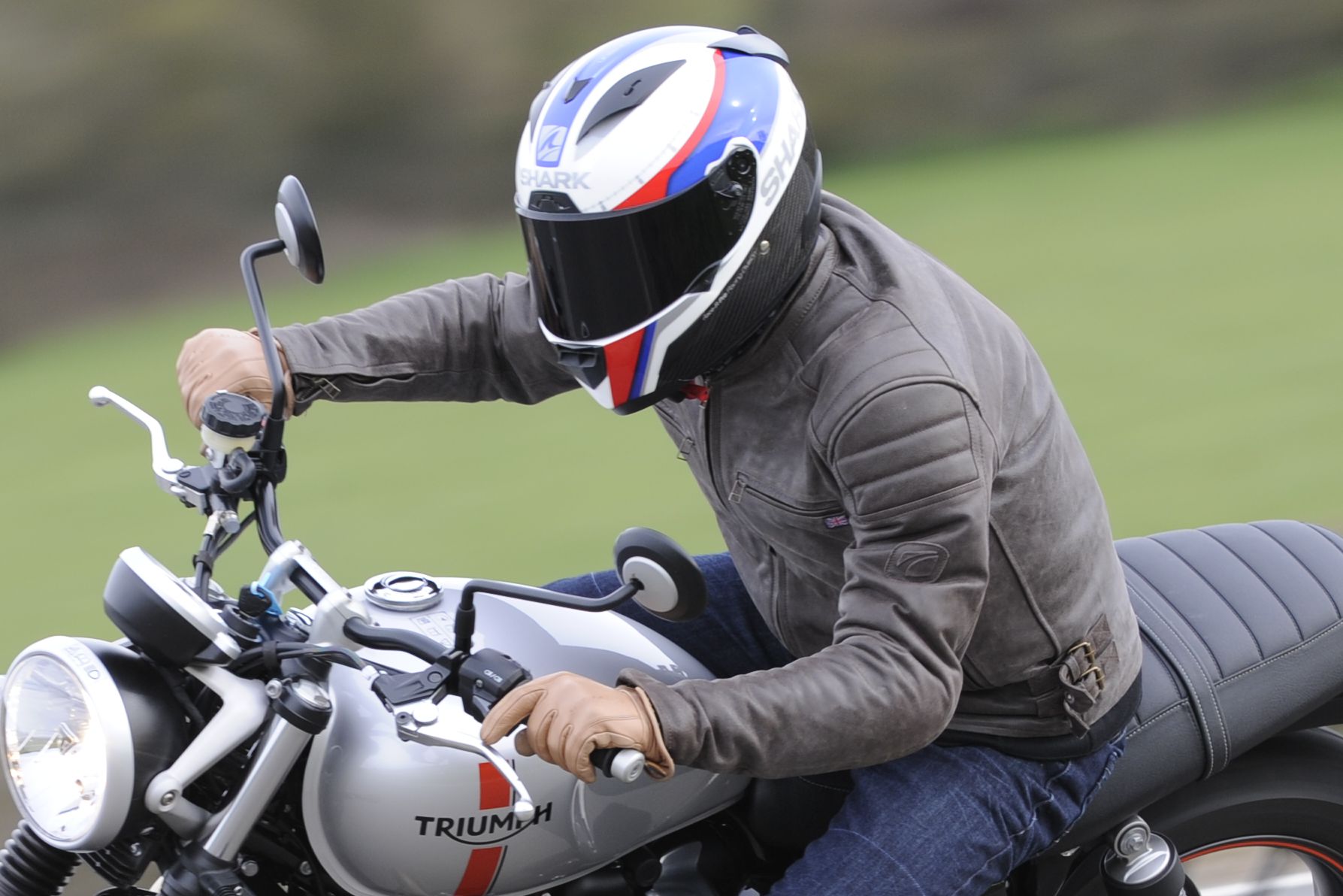A vibrant full-color photograph captures an outdoor daytime scene featuring a motorcyclist pivoting slightly to his left. The background is a blur of greenery and trees, suggesting a verdant setting. The motorcyclist, presumed to be a man, is decked out in protective gear: a distinctive helmet with a white, red, and blue design and a dark visor, branded with 'Shark', a gray jacket with pleats at the shoulders and biceps, tan gloves, and blue jeans. He is seated on a stylish Triumph motorcycle, identifiable by the black leather seat and the silver gas tank emblazoned with the Triumph logo, accented with a red stripe cutting through the "M." The motorcycle dashboard, headlights, and a rearview mirror peeking over his right shoulder are all visible. The framing of the photograph captures him from the thighs up, with the image cutting off the wheels of the bike. The overall ambiance combines the thrill of motorcycling with the serene clarity of a sunny day outdoors.